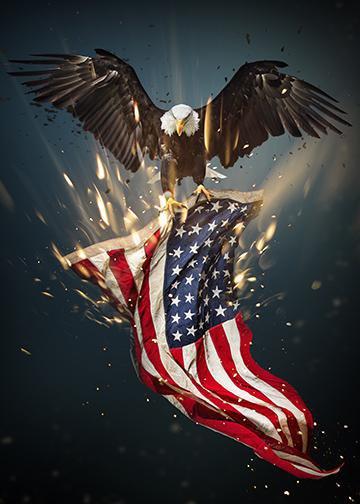This image is a vertically aligned rectangular piece of art, likely computer-generated, resembling a dramatic poster. It features a fierce bald eagle with a white head and yellow beak, soaring towards the viewer with its large brown wings spread wide. Its yellow claws grip the white border of an American flag, which billows downwards as if caught in the wind. The flag displays the stars just below the eagle's claws and the red and white stripes flowing gracefully. The eagle’s head is slightly tilted downward, enhancing its intense gaze. The background transitions from dark black at the bottom to dark blue towards the top, creating a deep, atmospheric effect. Accentuating the scene are bright, golden streaks or sparks around the flag, adding a dynamic sense of motion and energy. These luminous accents resemble flames, intensifying the image's dramatic impact.